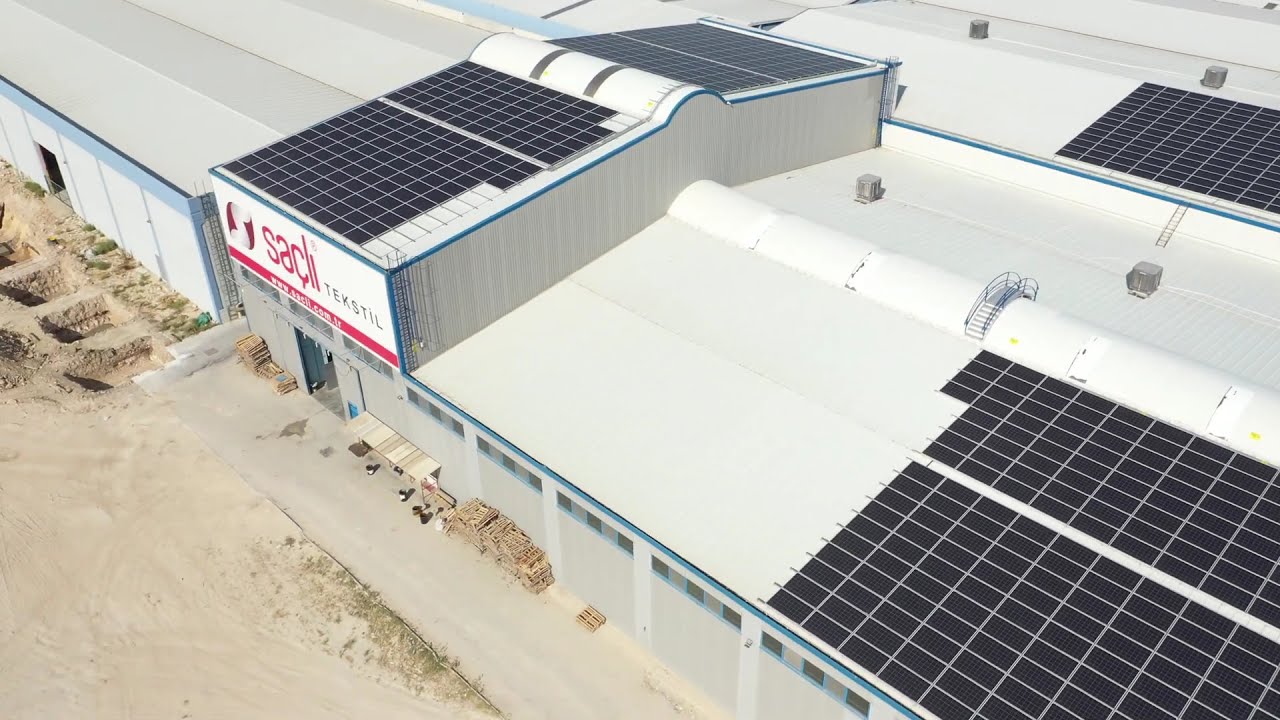This overhead photograph showcases a large, rectangular warehouse or industrial building, its white, flat roof running diagonally from the upper left to lower right of the image. Prominent on the roof are several elevated blocks of solar panels—four distinct sections can be identified, contributing to a substantial solar array. A notable feature on one of these elevated blocks is a white sign with a red bar at the base, displaying the letters "SACI" alongside smaller, unreadable text. The building itself features garage bay doors, two of which are open, revealing an interior likely used for storage. In front of the bays are stacks of boxes and pallets. The lower left foreground of the image reveals a paved driveway or parking area, suitable for trucks to load or unload cargo. Surrounding the entrance and driveway are sections of dirt or gravel, possibly indicating ongoing construction or heavy vehicle traffic.